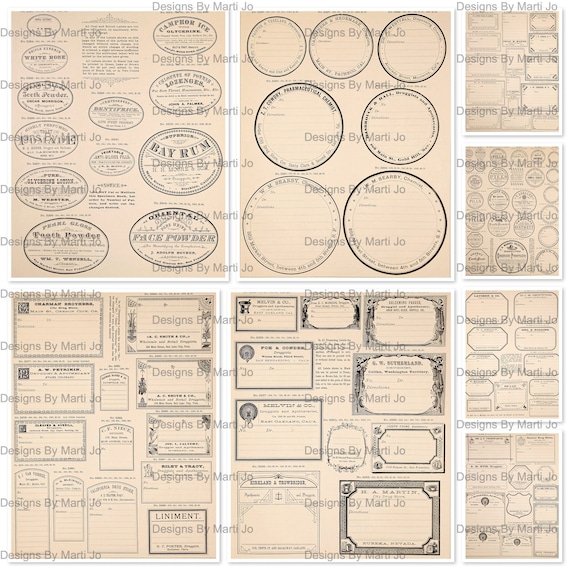The image displays an array of various design templates meticulously aligned in a grid format. Each set of designs, prominently watermarked with "Designs by Marti Jo" to ensure copyright protection, showcases potential layouts for labels or business cards. The designs feature a diverse selection of shapes including circles, ovals, squares, and rectangles, with each template varying in size and stylistic details such as borders and fonts. Scattered across the designs are discernible labels such as "Bay Rum", "Lozenges", "Camphor Ice", "Liniment", "Teeth Powder", and "Oriental Face Powder," suggesting tailored applications for different products. Despite some text being difficult to read, the intricate collection underscores Marti Jo's capability to create customized and professionally crafted business labels and cards.